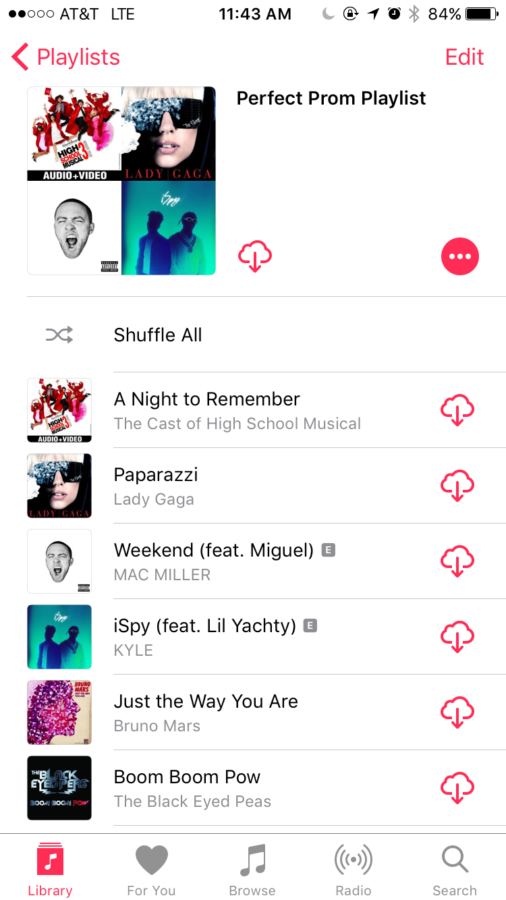The screenshot is taken from a cell phone, specifically showing a music playlist screen. 

In the upper left-hand corner, the display indicates that two out of five signal strength dots are black, signifying low signal strength, and it shows "AT&T LTE" as the network. Central at the top, the time is displayed as "11:43 AM," while the upper right corner reveals an 84% battery life remaining.

The following row includes navigation icons in red: a return arrow on the far left, the label "Playlists" in the center, and an "Edit" option on the far right.

Underneath, the screen is divided into two main sections. On the right-hand side, the text reads "Perfect Prom Playlist" with a red download symbol beneath it. Additionally, there is a red circle containing three white dots, indicating additional options. On the left-hand side, four thumbnail images represent the playlist content, suggesting that these are tracks suitable for DJing a prom. The thumbnails include "High School Musical 3," an image of Lady Gaga, and two other unspecified thumbnails.

Below this, a row labeled "Shuffle All" is present, allowing users to shuffle the entire playlist.

Subsequently, numerous rows present three columns each: the left column features album or track images, the middle column lists the song titles, and the right column holds a red download button for each track.

The listed songs begin with:

1. "A Night to Remember" by the cast of "High School Musical"
2. "Paparazzi" by Lady Gaga
3. "Weekend"
4. "I Spy"
5. "Just the Way You Are"
6. "Boom Boom Pow"

Finally, in the bottom left-hand corner, the "Library" tab is highlighted in red, indicating that the user is currently in the library section of the app.